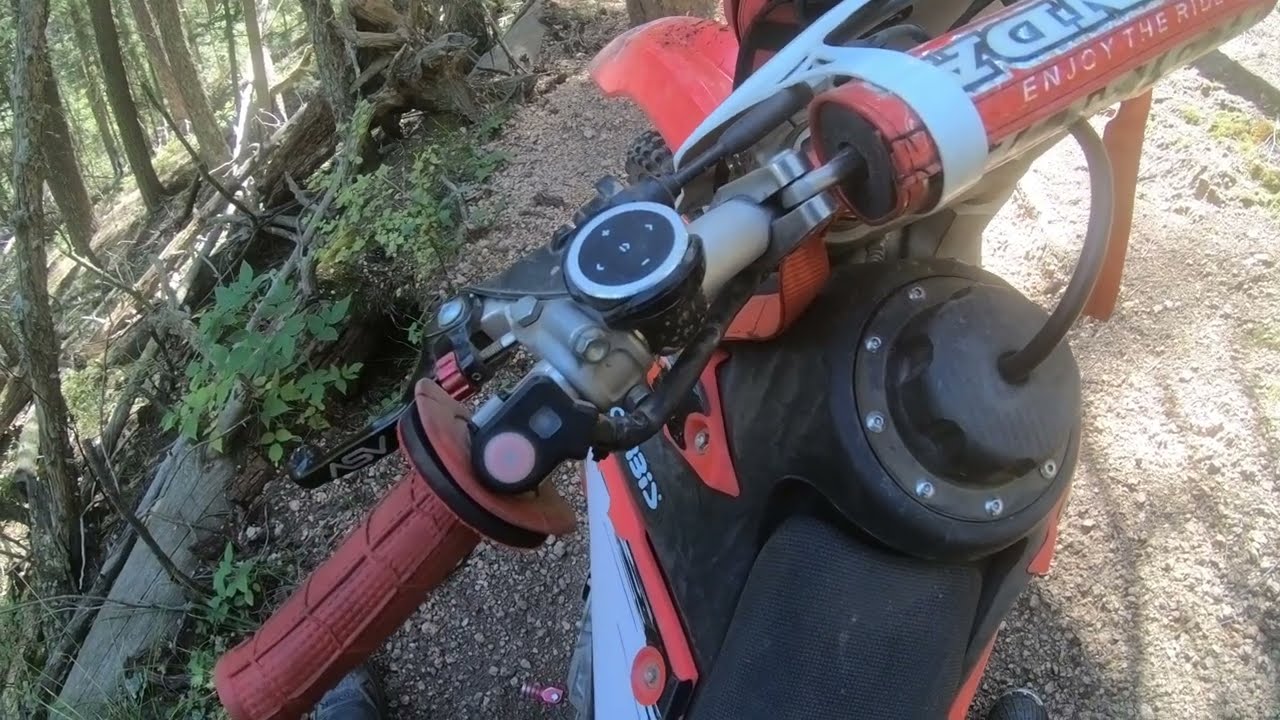This full-color photograph captures a scenic, daytime outdoor adventure in the woods, presented in a horizontally rectangular format without any border. At the forefront of the scene, a Honda dirt bike, prominently black and red with hints of white and orange, commands attention. The close-up perspective reveals intricate details: the left handlebar equipped with a black brake and red rubber grip, a black gas cap positioned near the handlebars, and a red foam padding emblazoned with the motto "Enjoy the Ride" in the bike's center. The sturdy black tire beneath exhibits deep grooves, suitable for the gravelly, clay-laden path it rests upon.

The surrounding milieu is a dense forest, abundant with an array of trees, some adorned with green leaves while others display bare trunks and branches. Mixed into the forest floor are patches of green weeds and fallen timber. Sunlight filters through the canopy, casting dappled shadows that add depth to the vibrant scene. While no rider is visible on the bike, the image suggests a paused moment of tranquil contemplation amidst nature's raw beauty. The viewer is left with the sense of sitting on the bike, perhaps ready to resume the journey along this serene woodland trail.